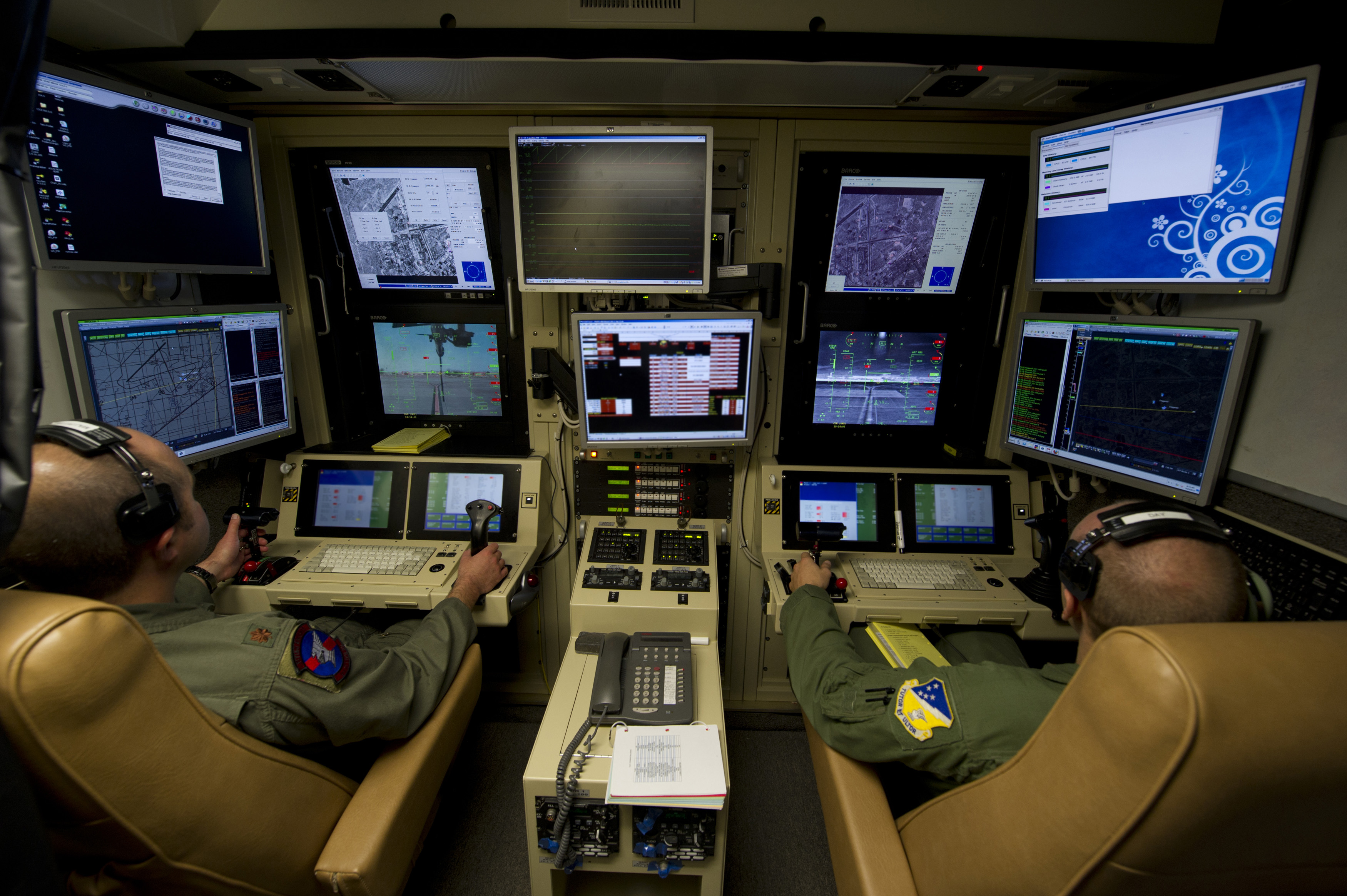In the image, two men dressed in military uniforms sit in brown, possibly leather, chairs equipped with armrests. They are inside a control center, which resembles a flight deck but without a window view. The room is filled with multiple computer screens: each man has a pair of side monitors displaying various software, and in front of them are vertically stacked screens—the bottom one seemingly used for navigating their simulation, possibly a flight simulator, showing a runway or technical aircraft information. Additional screens and equipment, including two smaller screens and keyboards, extend below their main displays. Both men are focused, gripping joysticks with both hands, and wearing headsets. Positioned centrally between them is a telephone alongside various other gadgets and a notebook. The wall behind them is lined with about ten different-sized monitors, displaying assorted information, contributing to the high-tech atmosphere of the control center.